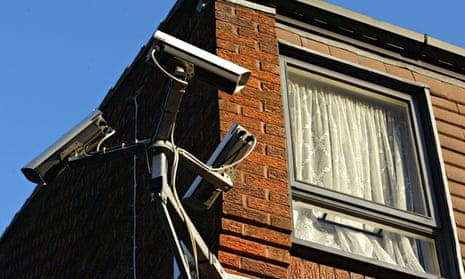The photograph captures the top corner of a red brick building, viewed from the bottom up. The building’s facade, illuminated by sunlight, prominently features a partially open window adorned with white or lacy beige curtains that obscure the interior. Alongside the window, slightly lower on the building’s wall, three security cameras are mounted, each pointing in different directions. These black and white cameras, with visible cabling, appear to be the focal point of the image. The background consists of a clear blue sky that frames the scene, emphasizing the structure's details and the security apparatus.